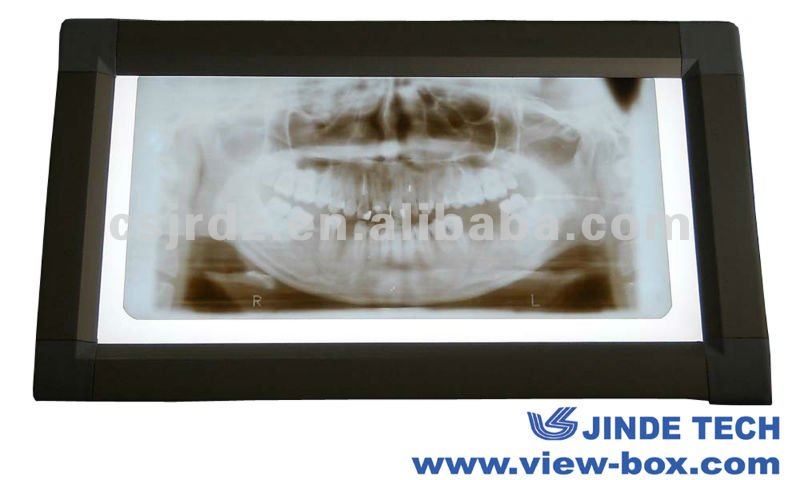This image depicts an x-ray of a person's jaw and teeth, displayed on an x-ray viewing machine designed to enhance visibility of the x-ray details. The x-ray itself, set within a thick black frame, reveals a clear, translucent image of the person's open mouth, showcasing the upper and lower jawlines along with numerous white teeth. Light emanates from behind the x-ray, illuminating the dental structures and accentuating various lines and streaks within the image. The letters 'R' and 'L' are visible on the left and right sides of the x-ray, respectively, indicating orientation. The edges of the frame are bordered with a bright light, with white strips visible on the left, right, and bottom sides. In the bottom right corner of the frame, there is a blue, oblong-shaped logo adjacent to the text 'JINDE TECH,' followed by the website 'www.view-box.com', marking the branding of the x-ray viewing machine. Additionally, a faint watermark reading 'asjrd2.en.alibaba.com' can be seen across the image, further suggesting its use as an advertisement for the viewing apparatus.